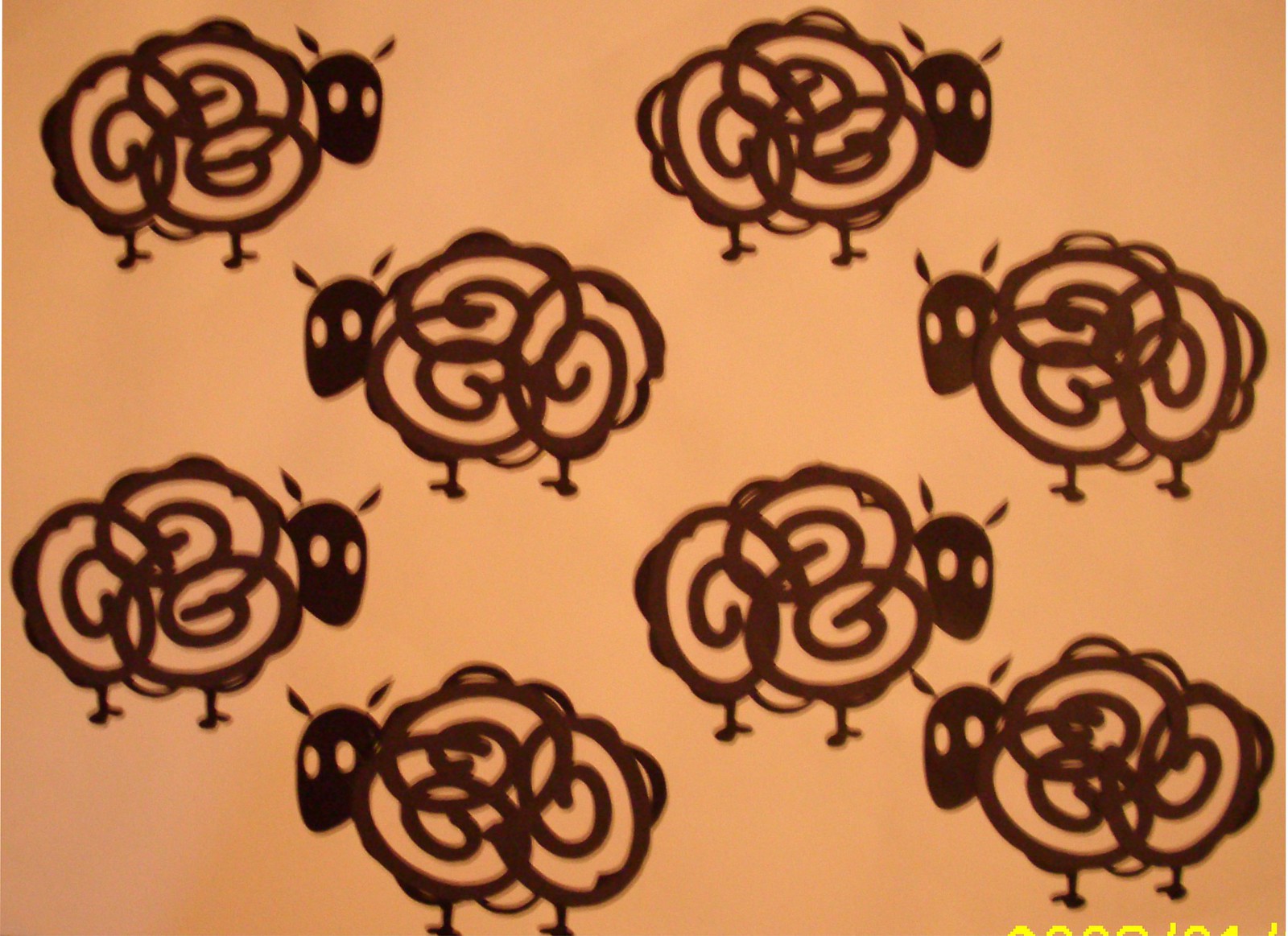The image displays a repetitive pattern featuring graphic depictions of sheep against a light, peachy-burnt orangey background. The sheep are arranged in four rows, each containing two sheep, with orientations alternating between right and left in each successive row. Each sheep is depicted with a black face characterized by white, negative space eyes and delicate, leaf-like ears positioned on top of their heads. The bodies, representing woolly coats, consist of a series of spirals or squiggles drawn in a dark, reddish-brown ink, while their feet are simple squiggle lines. The pattern evokes a tribal or tattoo-like aesthetic. In the bottom right-hand corner of the image, there's a hint of yellow lettering that appears cut-off. The overall composition presents a cohesive yet dynamic visual, where none of the sheep overlap but are perfectly spaced to create a seamless and orderly pattern.